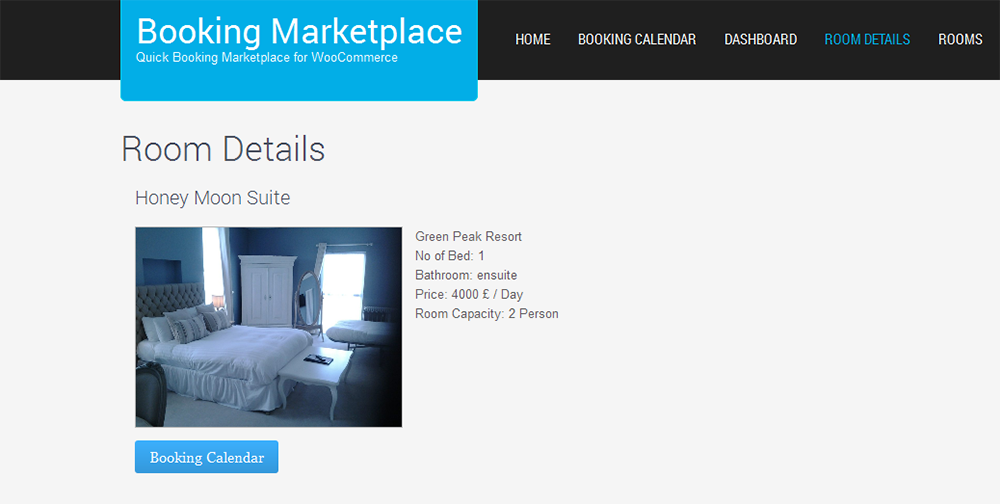The image displays a webpage from a website named "Booking Marketplace" specifically tailored for WooCommerce. At the top, a black navigation bar stretches across the screen. Towards the left within this black band, a blue rectangle showcases the website's name in large white letters, stating "Booking Marketplace," with a tagline beneath it reading "Quick Booking Marketplace for WooCommerce."

To the right within the black band, several menu options are listed in white text: "Home," "Booking Calendar," and "Dashboard." An additional menu option, "Room Details," is highlighted in blue, indicating the current selection with the final option "Room" also in white text.

Below the navigation bar, the page background is predominantly white. Centered in large black letters, the header reads "Room Details," followed by a subtitle in smaller letters that says "Honeymoon Suite." Below this text, a color photograph captures an opulent room featuring a neatly made bed adorned with a white cover and several pillows. In the background, the room includes several windows and a closet door, framing the scene.

To the right of the photograph, descriptive details about the room are listed: "Green Peak Resort," "Number of Beds: 1," "Bathroom: en Suite," "Price: £4,000 a day," and "Room Capacity: 2-person."

Beneath the photograph, a prominent blue rectangular button displays the text "Booking Calendar" in white letters, inviting users to explore booking availability.